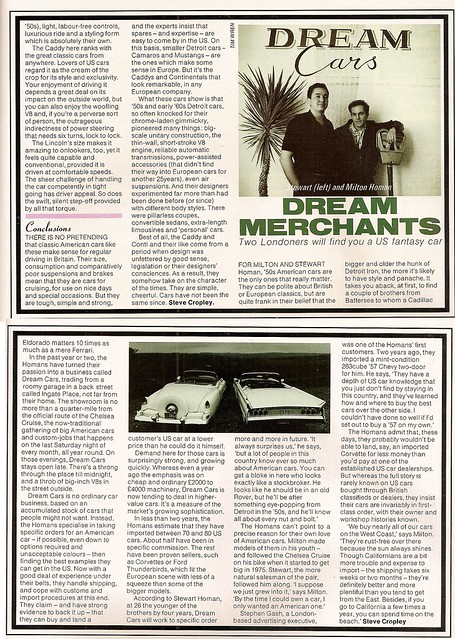The image depicts two pages of a dated magazine article titled "Dream Merchants: Two Londoners Will Find You a U.S. Fantasy Car." The article, written by Steve Cropley, features two men, identified as brothers Stuart and Milton Horton, standing side by side. Stuart is seen leaning against a parking meter while Milton stands before a backdrop with a palm tree. In the photographs at the top of the first page and bottom of the second page, vintage American cars like Cadillac convertibles from the 1950s or '60s with prominent fins and spare tires are showcased. The brothers' business, Dream Cars, is detailed within the article, revealing their passion for sourcing and providing classic American cars to enthusiasts. The article explains how they've established a showroom in Engate Place, near the Chelsea Cruise route in London, where each month, a gathering of American car lovers takes place. Amidst the throng of big V8 engines, Dream Cars remains open late, catering to the influx of visitors drawn by the spectacle of these luxuriant vehicles.